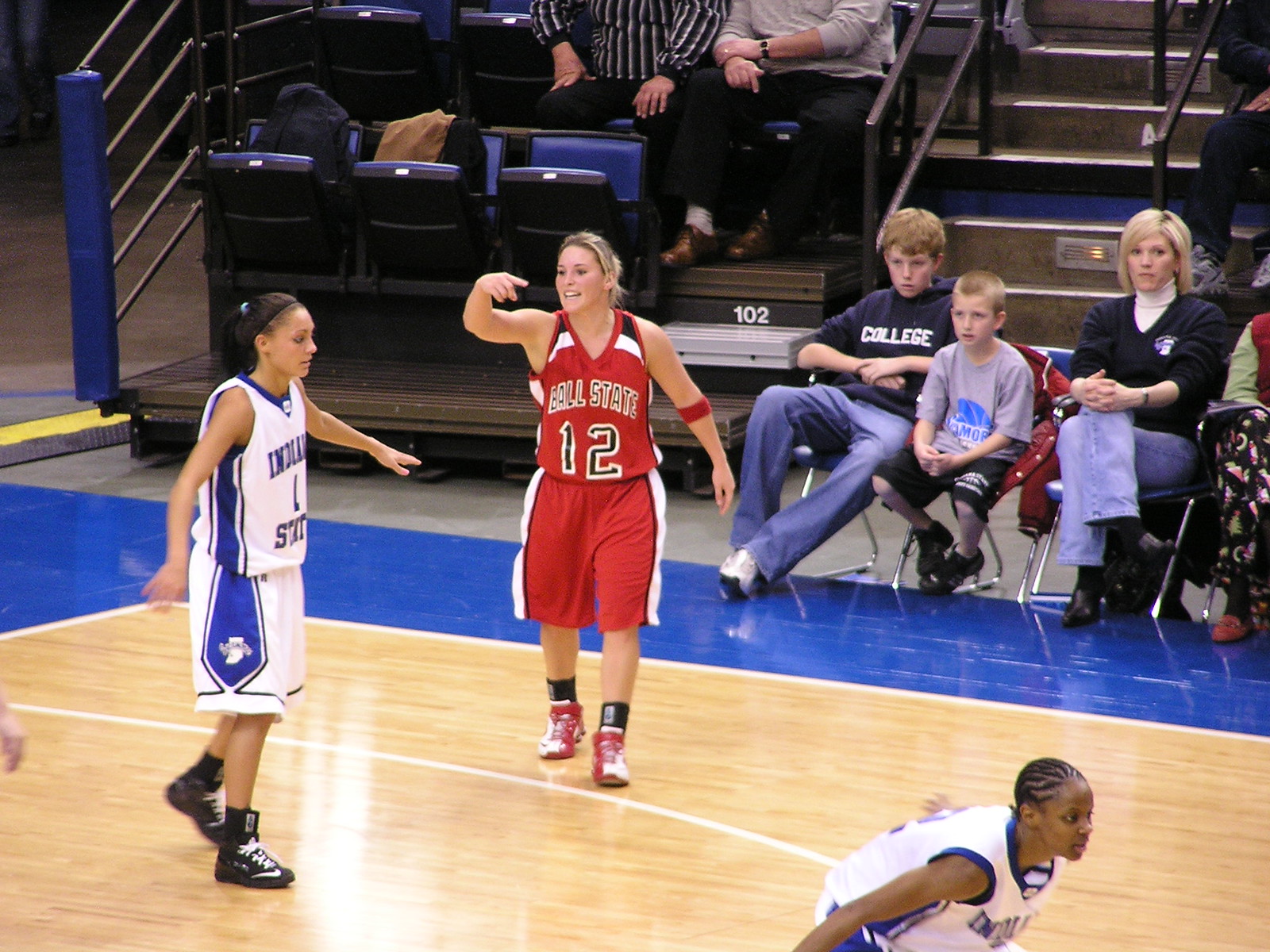The photograph captures an intense moment during a women's college basketball game between Indiana State and Ball State, played on a polished, light brown wooden court with blue and white markings. The central focus is on three players: a Ball State player, number 12, who has blonde hair and is prominently positioned in her red and white jersey with her hand gesturing towards the sidelines, possibly communicating with a coach or teammate. To her right, an Indiana State player, wearing jersey number 1 in white and blue, has her arms outstretched as if in preparation for defense. Another Indiana State player is bent over, ready to guard an opponent. The background reveals a mix of spectators, including children and adults, seated courtside on folding chairs and in the bleachers. The arena atmosphere is lively, with fans attentively watching the unfolding action.